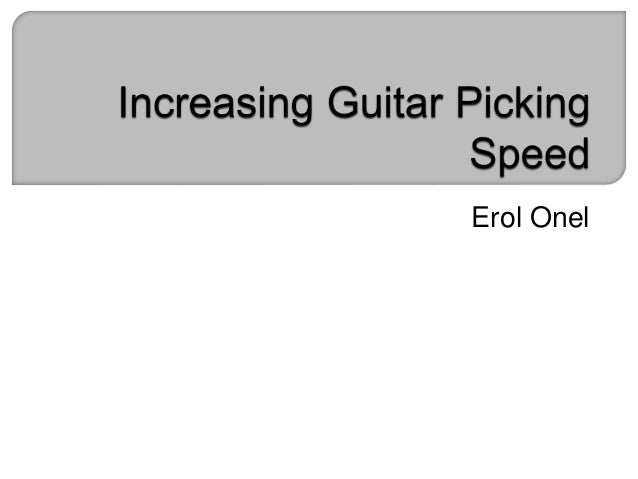The image is a simple and plain photograph of a rectangular sign, likely taken from a book or a manual. The top portion of the image features a light gray background with rounded corners on the top left and bottom right. The black text on the gray background reads "Increasing Guitar Picking" on one line and "Speed" directly underneath it. The bottom portion of the image is plain white, and below the gray section, in black lettering, it says "EROL ONNEL." There are no additional elements such as a frame, dates, locations, or pictures, and it exclusively features text on a clean, two-tone background.